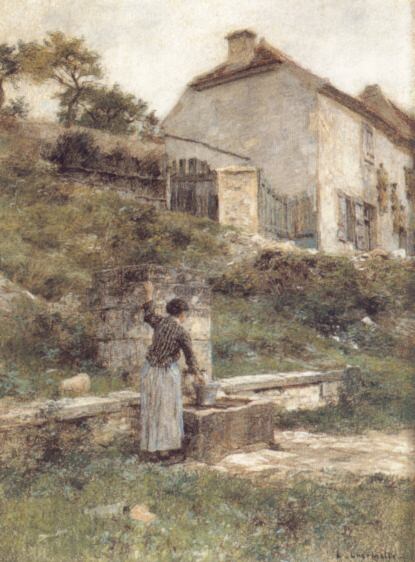The image appears to be a reproduction of an oil painting with a muted color palette dominated by greens, browns, and grays. It features a woman prominently in the foreground, dressed in a long white skirt and a darker colored checked shirt with long sleeves. She stands beside a knee-high rock fence, with her right hand on a silver-gray bucket that might contain water and her left hand raised, possibly touching the fence. The woman has dark hair and appears focused on her task, which seems to involve working with the bucket, possibly pumping water.

The background of the scene includes a house or a stucco-type building situated on a hill, with a fence along its right side and trees to its left. The sky above is cloudy and gray, enhancing the overall muted tone of the painting. Brush and vines can be seen in front of the house, adding to the depiction of an old-fashioned, rustic setting. The landscape appears slightly slanted, contributing to a sense of depth and historical ambiance in the painting.